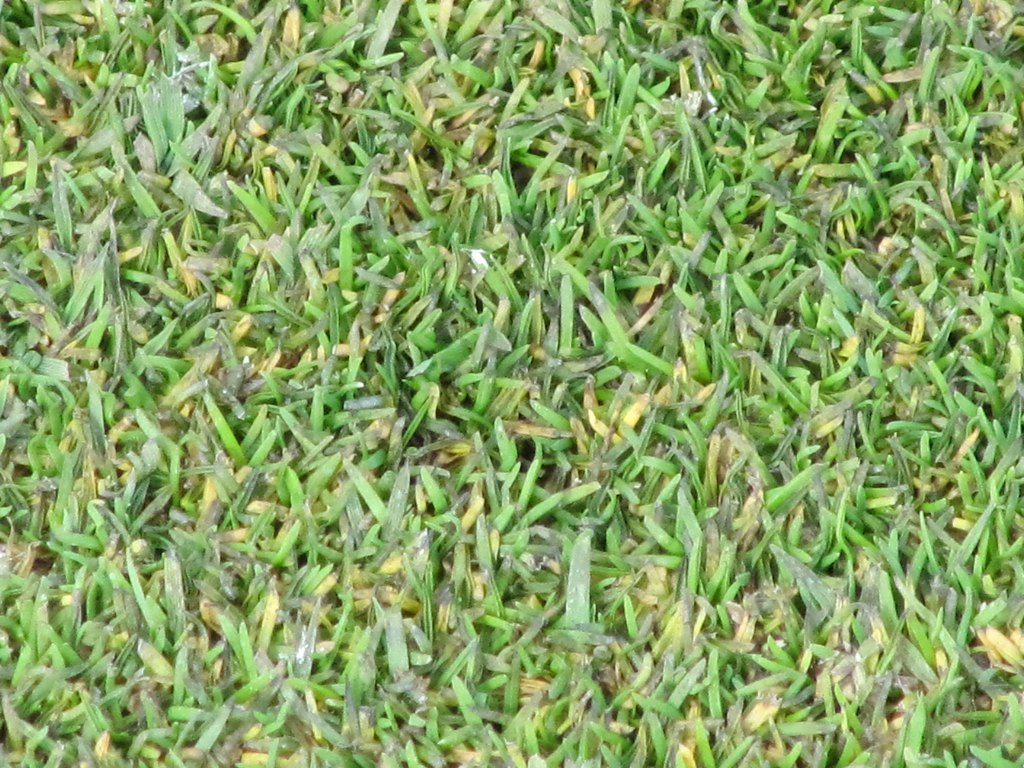The image is an up-close, horizontal photograph of neatly trimmed grass, displaying a diversity of colors and details. The grass blades dominate the entire frame from left to right and top to bottom, with no other objects or text present. The central section of the image features bright green blades, while the left-hand side shows a varied mix of light and dark green blades. The bottom right corner has blades extending in multiple directions, with some pointing left and others right. Throughout the image, there are different shades of green, including dark green, light green, grayish-green, and even specks of lime green. There are also occasional yellow and white blades of grass interspersed. At the top, the blades appear slightly longer, showcasing an array of fresh, vibrant colors without any other background elements like sky or distant objects. The photograph vividly captures the texture and variety within the grass, highlighting the intricate details of each individual blade.